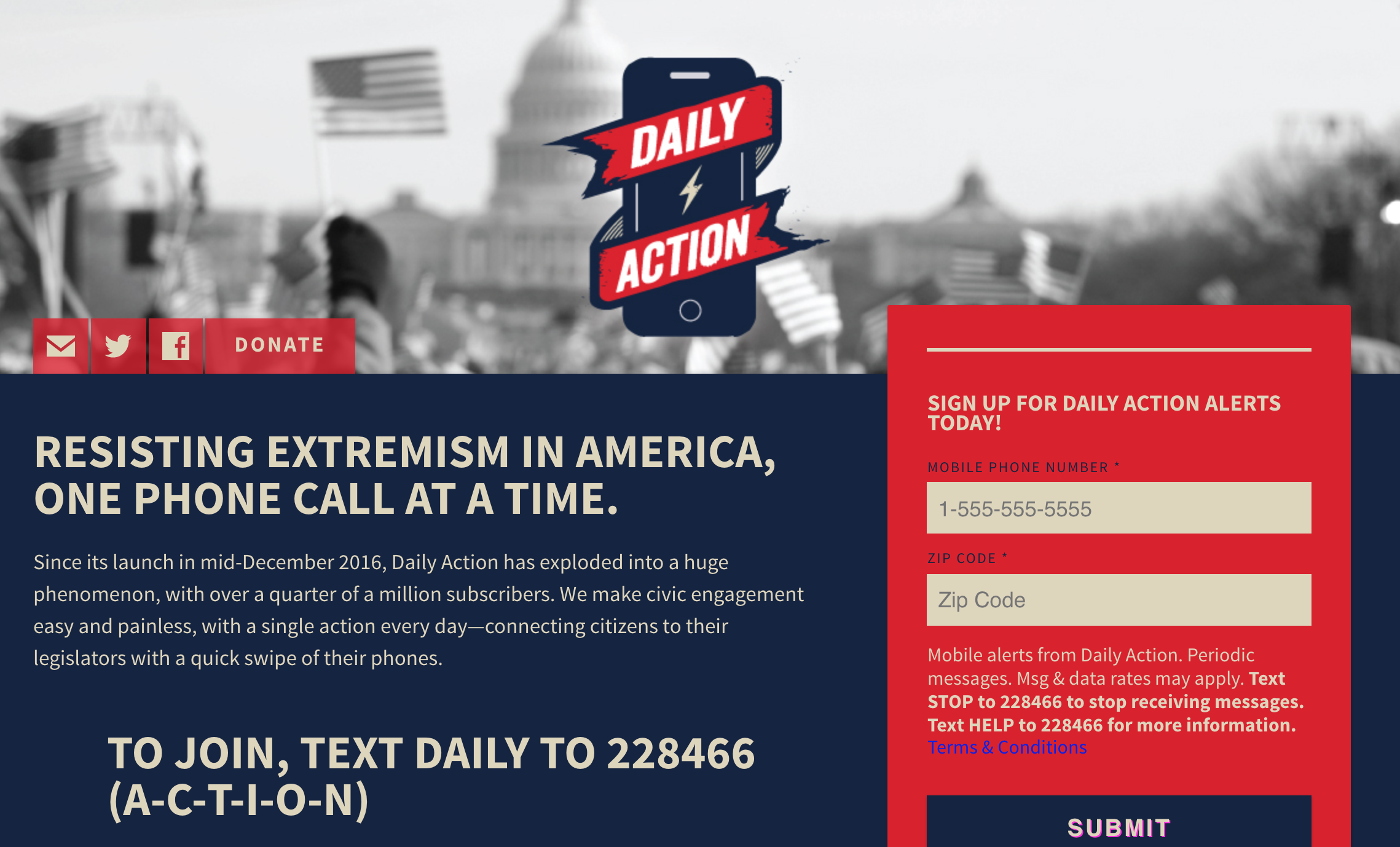A black and white screenshot captures a scene set against the backdrop of the U.S. Capitol, prominently featuring the White House and American flags waving as if during a presidential speech. The central focus of the image is a bold banner with the text "DAILY ACTION" flanked by a mobile phone icon and a lightning bolt. Below this, a series of social media icons for email, Twitter, Facebook, and a bold "DONATE" button are visible. 

On the right side of the banner, there is a sign-up form inviting users to receive daily action alerts by entering their mobile phone number and zip code. On the left, a bold, capitalized heading reads, "RESISTING EXTREMISM IN AMERICA, ONE PHONE CALL AT A TIME." Beneath this heading, a yellowish text on a blue background provides details: 

"Since its launch in mid-December 2016, Daily Action has exploded into a huge phenomenon. To join, text DAILY to 2284 ACTION."